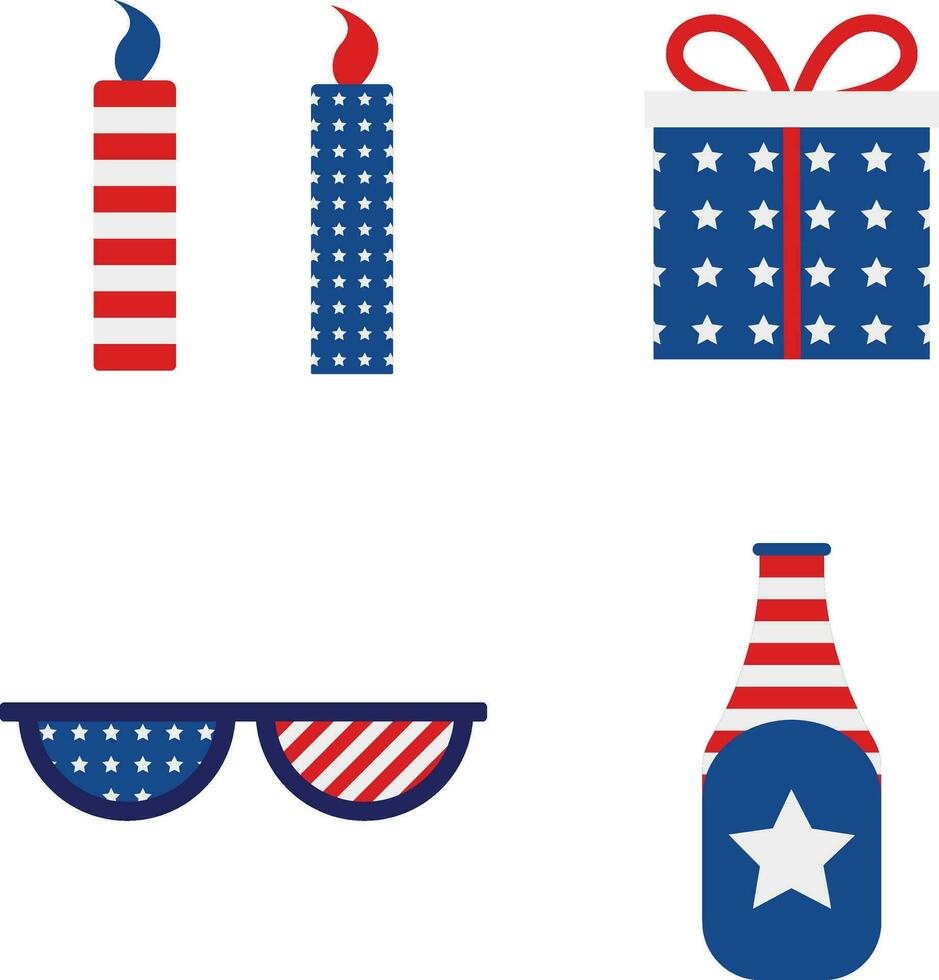The image showcases an assortment of items detailed in the patriotic colors of red, white, and blue, styled in a thematic tribute likely for a 4th of July celebration. On the left side of the image, two candles stand prominently: one candle features a layered design in red, white, and blue with a distinctive blue flame, while the adjacent candle is red with white stars set against a blue background, topped with a red flame. To the right of these candles, a gift box wrapped in blue paper adorned with white stars is visible, accentuated by a red bow.

Below the two candles are a pair of novelty glasses framed in blue. The left lens is designed with blue and white stars, whereas the right lens showcases red and white stripes. Further right, there is a patriotic-themed bottle with a blue top, transitioning into red and white stripes down the body, and concluding with a blue bottom highlighted by a singular white star. Each item collectively reinforces the celebratory tone and theme commonly associated with American patriotic holidays, particularly the 4th of July, by incorporating elements reminiscent of the United States flag.